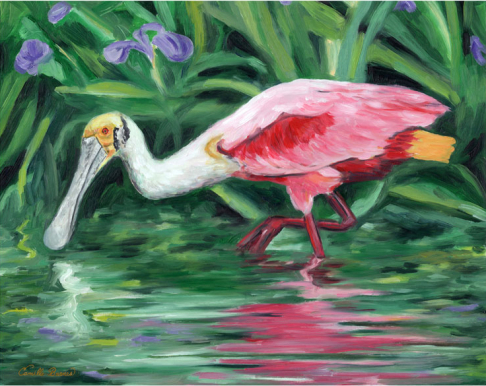This image is a detailed watercolor painting in landscape orientation, featuring a close-up of a roseate spoonbill, a tropical bird. Centered in the image, the spoonbill stands in shallow, greenish water with one pink, clawed leg holding it up and the other leg bent upwards. The bird is depicted in profile, with its white head and neck adorned with a splash of gold near the eyes. It has a long, gray, spoon-shaped bill dipping towards the water, and its eyes are tinged with shades of pink or red. The spoonbill's body primarily showcases pink feathers mixed into the surrounding water and foliage, creating a harmonious blend of colors. The background reveals lush, green, blade-like leaves interspersed with small purple flowers. The reflections of the bird and the plants are visible in the water, enhancing the painting's intricate detail and vivid palette.